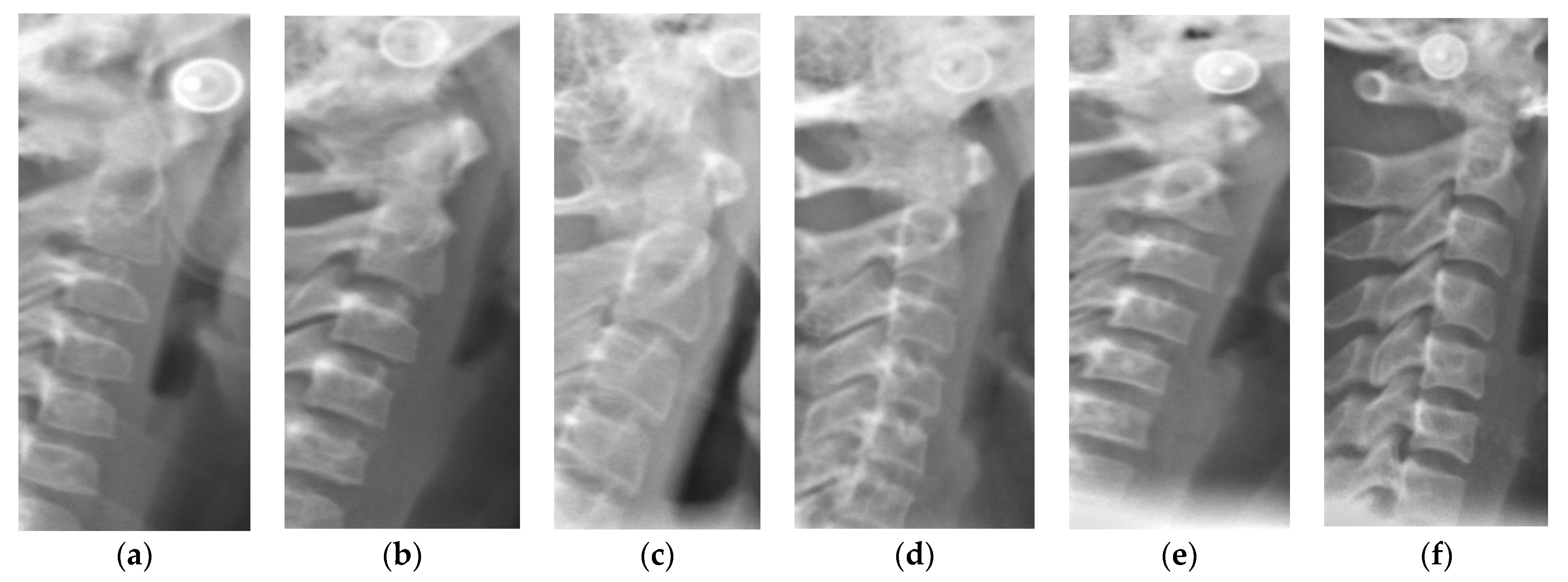The image features six black-and-white x-ray photographs of spinal columns, labeled A through F in parentheses at the bottom of each image set against a white background. Each x-ray displays a different spine, highlighting the vertebrae, with notable differences in the condition of the spinal discs. Some x-rays reveal abnormalities such as herniated discs or missing cushioning. Particularly, the x-ray labeled C appears the most abnormal, while E and possibly A seem relatively normal. At the top of each x-ray, there is a white circle with a small dark circle inside, consistently positioned across all six images.